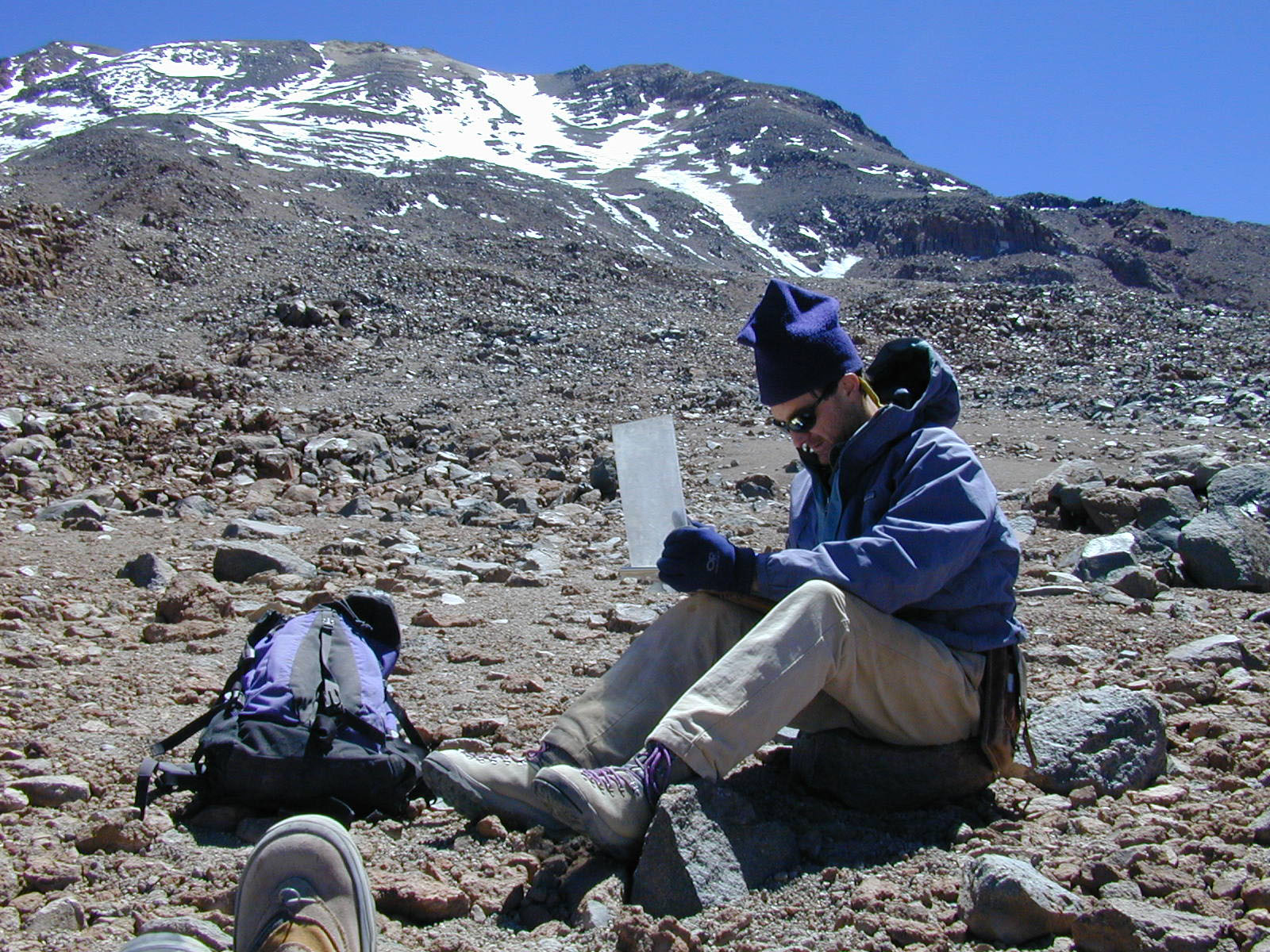The photograph captures a hiker taking a momentary rest during his ascent up a rugged, rocky mountain. The man, clearly dressed for a cold-weather hike, sits on a large gray rock surrounded by a mixture of dirt, gravel, and stones at the base of the mountain. His attire includes a light blue parka, beige khaki pants, tan hiking boots, a navy blue beanie, gloves, and sunglasses, suggesting harsh weather conditions at higher altitudes. To his left lies a blue and black hiking backpack—essential for his adventure.

He appears to be examining a rectangular piece of paper, potentially a map or notes, as he plans his next move. In the bottom left corner of the image, the tops of someone else's shoes, presumably those of the photographer, are visible, indicating they are also seated, their legs crisscrossed.

The mountain backdrop transitions from the rocky base where the man rests to snowy patches further up, emphasizing the increasing elevation. Above the mountain, the sky is a clear, medium blue with no clouds in sight, signifying a crisp, clear day ideal for hiking. The serene, expansive mountain scenery hints that the summit is not far off, adding to the sense of adventure and anticipation in the image.